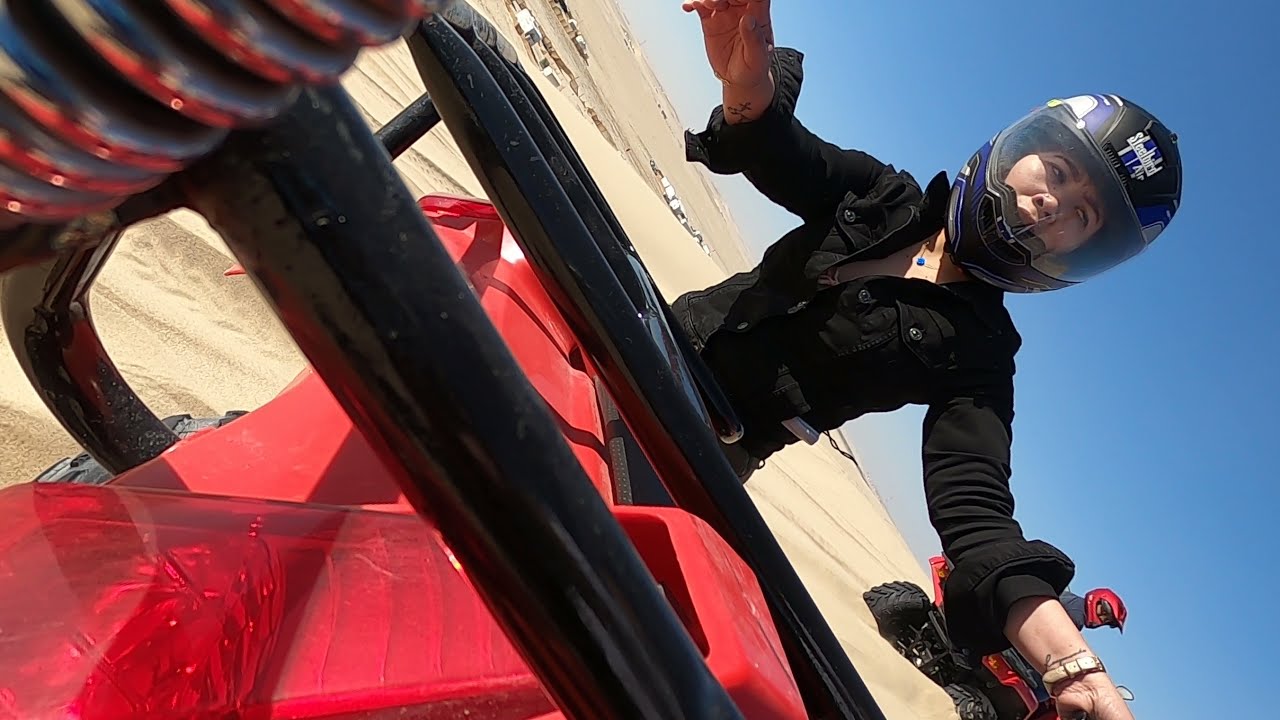This tilted photograph captures a dynamic desert scene featuring multiple ATV riders. Dominating the image is a woman at the center, wearing a long-sleeved black top and a black helmet with white text, though the text is unreadable. Her black and blue helmet partially obscures her face. She navigates a red ATV with black handlebars, and her arms are outstretched, gripping the controls. The desert terrain beneath is beige sand, marked by tire tracks. In the bottom right, another ATV rider, wearing a red helmet and black shirt, turns back to glance at the woman. The background shows an expanse of sand under a clear blue sky, with a makeshift parking area with several cars parked on the sandy surface. The photo is tilted sideways, adding a sense of action and movement to the scene.